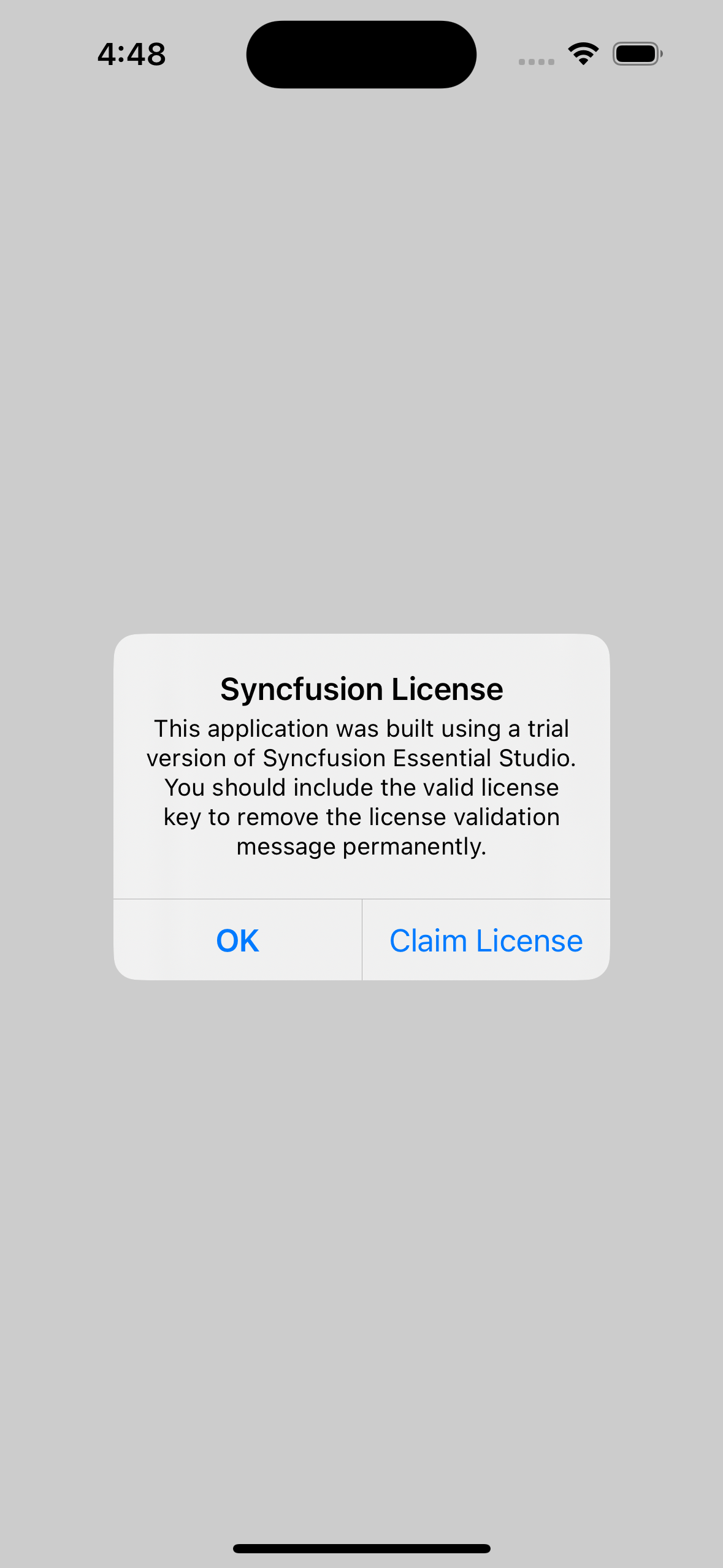The image displays a mobile application interface. At the top of the screen, the status bar reveals it is 4:48. The status bar includes icons for three dots, Wi-Fi connectivity, and battery level, albeit obscured by a dark oblong shape. The main background is predominantly a blank white-grey, providing a sharp contrast to a centrally placed lighter grey box. This box contains a message stating, "Syncfusion License: This application was built using a trial version of Syncfusion Essential Studio. You should include the valid license key to remove the license validation message permanently." At the bottom of this notification are two buttons labeled "OK" and "Claim License," both with text in blue.